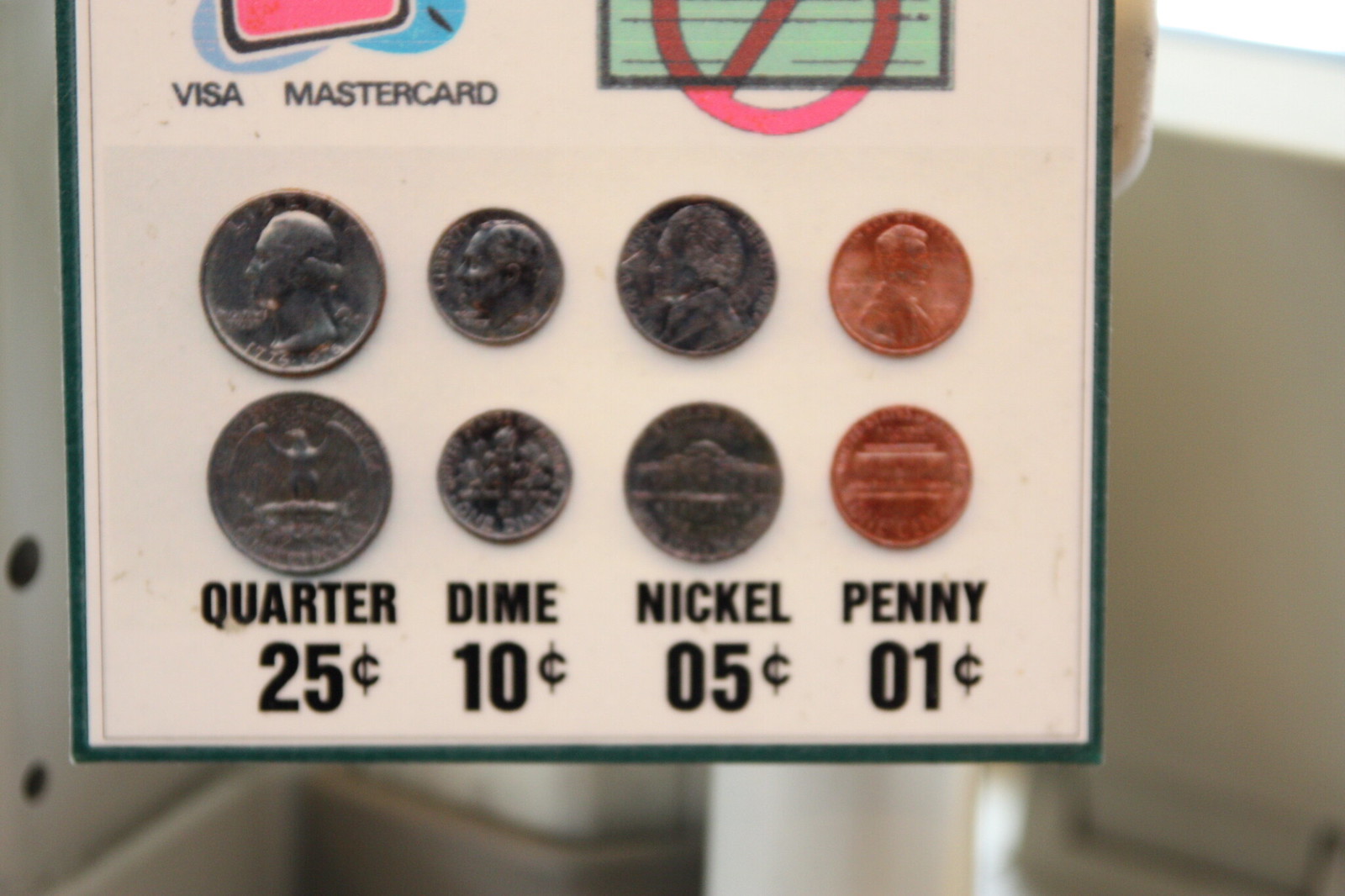This color photograph captures a sign with a white background rimmed by a green frame. At the top of the sign, the words "Visa" and "MasterCard" are partially visible, arranged on a white background in black letters. To the right of this text, there's an illustration of a credit card, presented in red with a black outline and blue accents. Adjacent to the credit card, a green check mark, detailed in black ink, is crossed out by a red circle and line, symbolizing a prohibition.

At the bottom of the sign, there's a detailed depiction of American coins, arranged in rows: two quarters, two dimes, two nickels, and two pennies, each showing their front and back sides. Text beneath each coin identifies them and their values in black lettering on the white background - "quarter, 25 cents," "dime, 10 cents," "nickel, 5 cents," and "penny, 1 cent." The quarters, dimes, and nickels are silver-colored, while the pennies are bronze. The sign is affixed at the lower left corner with black screws or nails, adding to its utilitarian appearance.